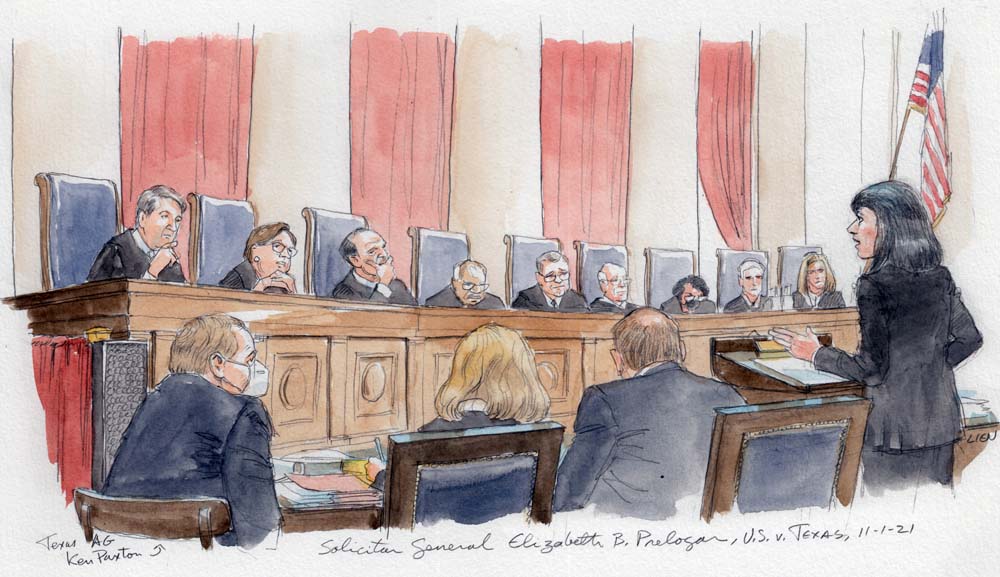The detailed artist’s rendering depicts a solemn courtroom scene inside the U.S. Supreme Court. Beige walls serve as the backdrop, adorned with long, plush red drapes covering the windows. On the far right, the red, white, and blue American flag stands prominently. The focal point of the painting is the grand wooden bench that extends across the scene, behind which sit the nine Supreme Court justices dressed in traditional black robes. Their tall, blue chairs add a sense of authority and gravitas.

In the foreground, a woman with long black hair, dressed in business casual attire, delivers an impassioned speech from the podium. The caption identifies her as Solicitor General Elizabeth B. Prelogar, advocating in the case of U.S. v. Texas (11-121). Seated nearby are various figures, including a blonde-haired woman and a dark-haired man. A particular point of interest is the person wearing a mask, identified by an arrow as Texas Attorney General Ken Paxton.